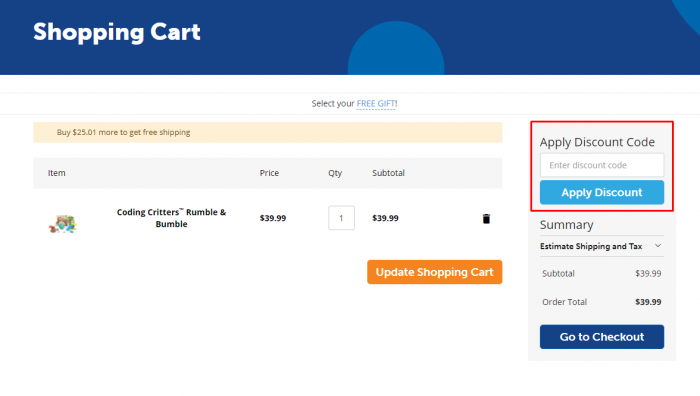A detailed caption for the image could be:

"This image depicts a screenshot from an online shopping cart, viewed on a mobile device. At the top of the screen, 'Shopping Cart' is prominently displayed in white text against a navy blue background. The navy background features a lighter blue semi-circle in the middle and a small lighter blue corner in the top right. Below this header, there is a section labeled 'Select your free gift,' with 'Free Gift' written as a clickable blue link. 

Further down, a tan rectangular box informs the user that they need to 'Buy $25.01 more to get free shipping.' Beneath this notification, there is an item listed: 'Coding Critters Rumble and Bumble,' priced at $39.99. The quantity is set to one, making the subtotal also $39.99. Adjacent to this information is a black trash icon for removing the item from the cart.

Additionally, there is an orange button labeled 'Update Shopping Cart.' Over on the right side, a red rectangle highlights the field for entering and applying a discount code, with instructions to 'Enter Discount Code' and 'Apply Discount Code.' At the bottom of the screen is a button labeled 'Go to Checkout.'"